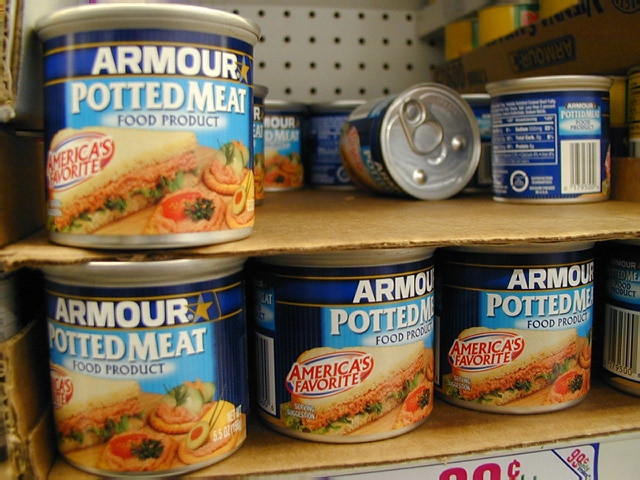Displayed on a grocery store shelf, this image showcases the world-famous Armour Potted Meat Food Product. The front of the shelf is adorned with a blue-bordered sticker indicating the price, which is 99 cents in pink font. Positioned within a brown cardboard box with its front cut off, the cans are stacked in both horizontal and vertical layers, resting on two tiers of cardboard separators. The bottom layer features three cans, while the top tier holds six or seven cans, with one can notably lying on its side, revealing its pull tab.

Each silver can is labeled with Armour's distinct blue branding, accented by a gold star. The cans boast the phrase "America's Favorite" in red print above an appetizing photo of a sandwich topped with potted meat. Additional images on the label depict the product served in various appealing ways, such as on white bread with lettuce, or on crackers garnished with avocado, tomato, olives, parsley, and cucumber slices. This detailed display unmistakably highlights the Armour Potted Meat food product, prominently positioned for an enticing purchase at an affordable price.